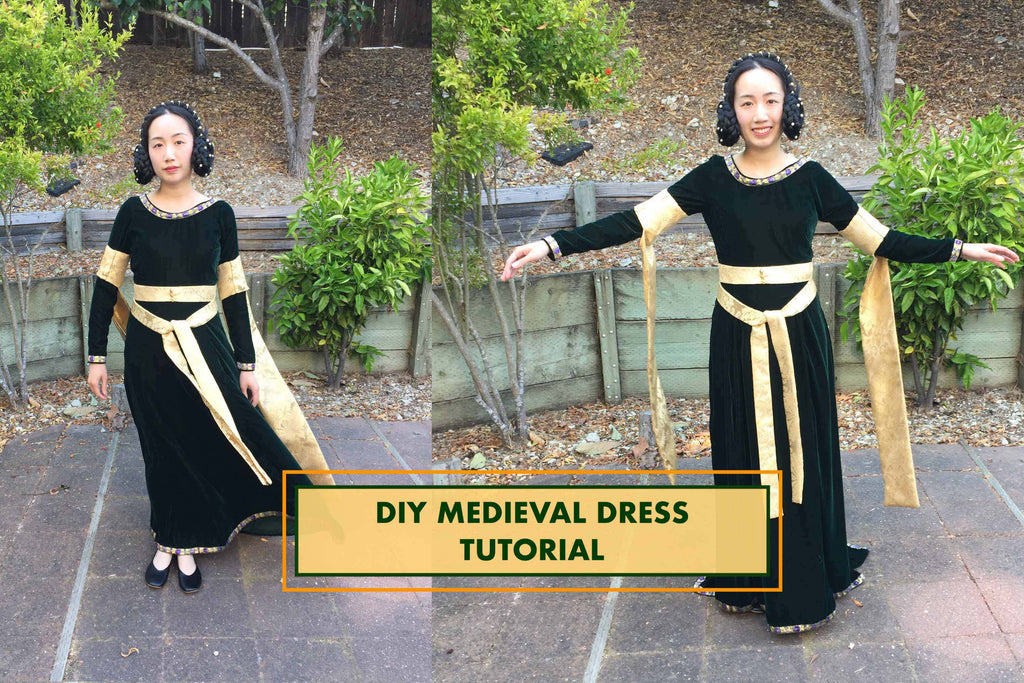The image, titled "DIY Medieval Dress Tutorial" in bold, all-caps green letters on a light brown rectangle outlined in green, features two side-by-side photos of an Asian woman wearing a black dress with intricate gold wraps around her waist and arms. The woman, who has her black hair styled in braided circles covering her ears and adorned with gold decor, is standing on a sidewalk against a background of a short wooden retaining wall, dirt, leaves, bushes, and trees. In the left photo, she stands with her arms down and a neutral expression, while in the right photo, she smiles and extends her arms outward. She is also wearing black flat shoes. The vibrant background adds a natural, rustic element to the tutorial theme.